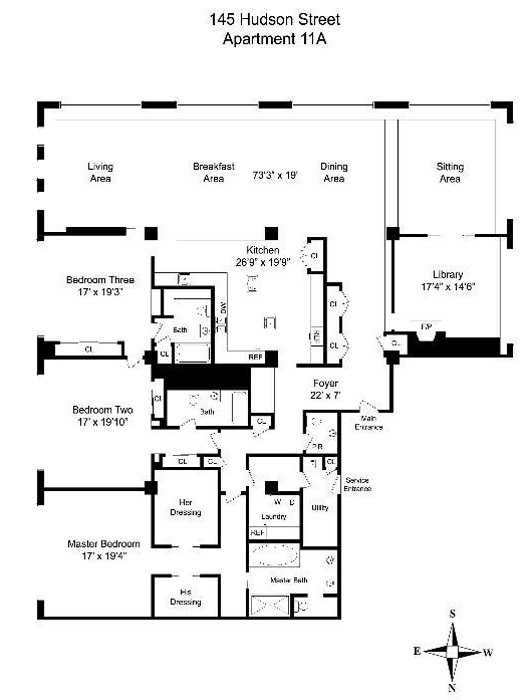Architectural drawing of Apartment 11A at 145 Hudson Street. This expansive, single-floor residence exudes luxury and intricacy in its design. Upon entering through the main entrance, guests are welcomed into a grand foyer measuring 22 feet by 7 feet. Adjacent to the foyer is a spacious kitchen, which seamlessly flows into a large living area, breakfast nook, and dining space—creating a harmonious open-concept environment ideal for both daily living and entertaining.

In proximity to the living and breakfast areas are three bedrooms: Bedroom Three, Bedroom Two, and the Master Bedroom. The Master Bedroom is particularly lavish, featuring separate his and her dressing rooms, a master bathroom, and a laundry and utility room for added convenience.

On the opposite side of the kitchen and foyer, the apartment boasts a library and a cozy sitting area, perfect for relaxation or study. The layout also includes a designated living room area. 

A small compass located at the bottom of the blueprint indicates cardinal directions, albeit in an unconventional manner with South positioned at the top and North at the bottom. This meticulous and thoughtful design reflects both style and comfort in the heart of this high-end apartment.